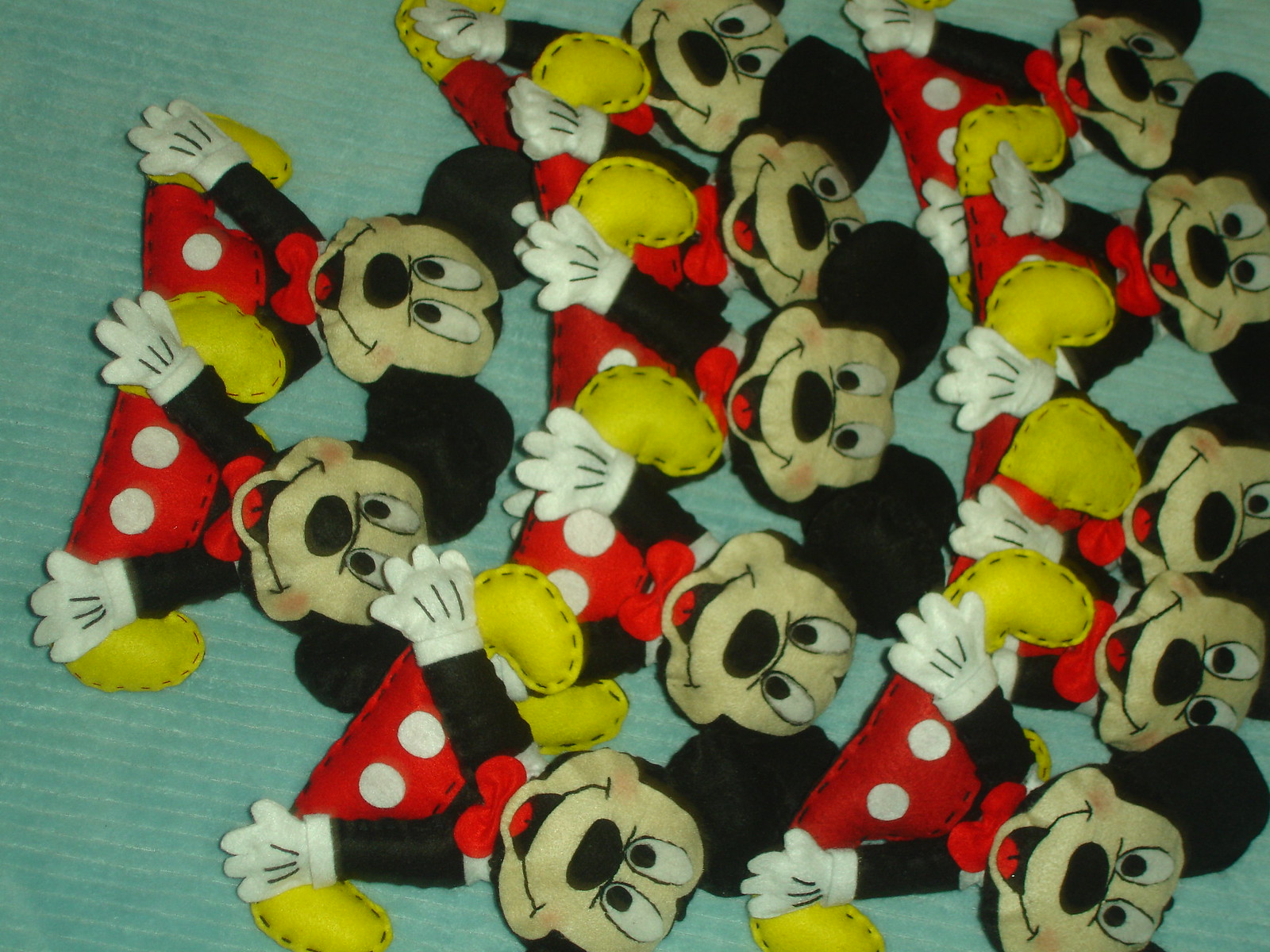This image features a collection of small, hand-stitched Mickey Mouse figures, each meticulously crafted from printed fabric, potentially cotton, and stuffed with polyester fiber batting. The Mickey Mouse figures, easily identifiable by their iconic black ears, open-mouthed smiles, and pale beige faces, are adorned with red shorts embellished with white buttons, white gloves, and yellow shoes. Each figure is positioned in a unique sitting pose, with legs spread apart and hands placed in front of them in a triangular formation. 

The setup showcases 12 identical Mickey Mouse figures, systematically arranged in three rows: the first two rows contain five figures each, while the bottom left houses the remaining two. All the figures are uniformly oriented with their heads pointed to the right and hands and feet towards the left. They rest upon a background that could be a light bluish-teal, powder blue fabric, or striped pale green surface, contributing to the whimsical and organized display. The craftsmanship suggests they could be used as patches, ornaments, or small plush toys.